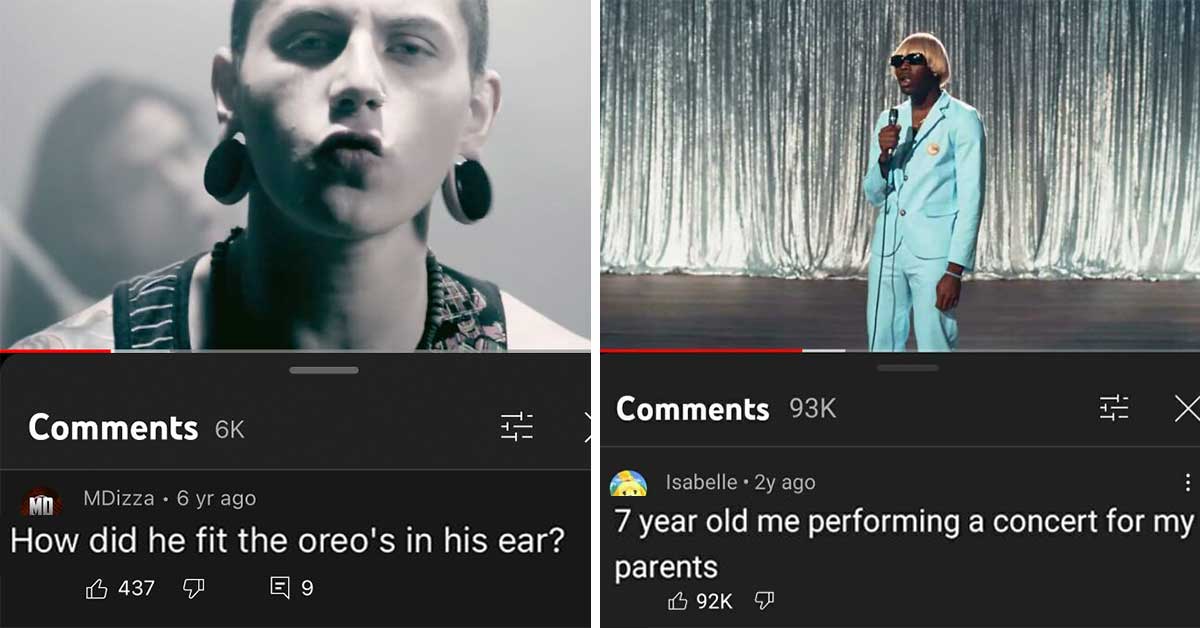The image is split into two columns with distinct photos and comment sections. 

In the left column, there is a picture of a music artist, who is white and wearing extremely large earrings in both ears. Below this photo, there is a vibrant comment section boasting 6,000 comments. The highlighted comment comes from a user named "MDESA" who posted six years ago. The comment humorously questions, "How did he fit the Oreos in his ear?" and has garnered 437 likes, though there is an option to dislike without any current tally.

In the right column, the second photo features Tyler, the Creator. He is wearing shades, a blonde wig, and a light blue suit and pants while standing on a stage adorned with a silver showcase curtain in the backdrop and what appears to be a tiled or wooden floor. The comment section for this photo is substantially more active with 93,000 comments. The top comment is from a user named "Isabel," posted two years ago, nostalgically stating, "Seven-year-old me performing a concert for my parents." This comment has received an impressive 92,000 thumbs-up, with the dislike option present but not quantified. Unlike the first photo, this one does not have its own dedicated comment section.